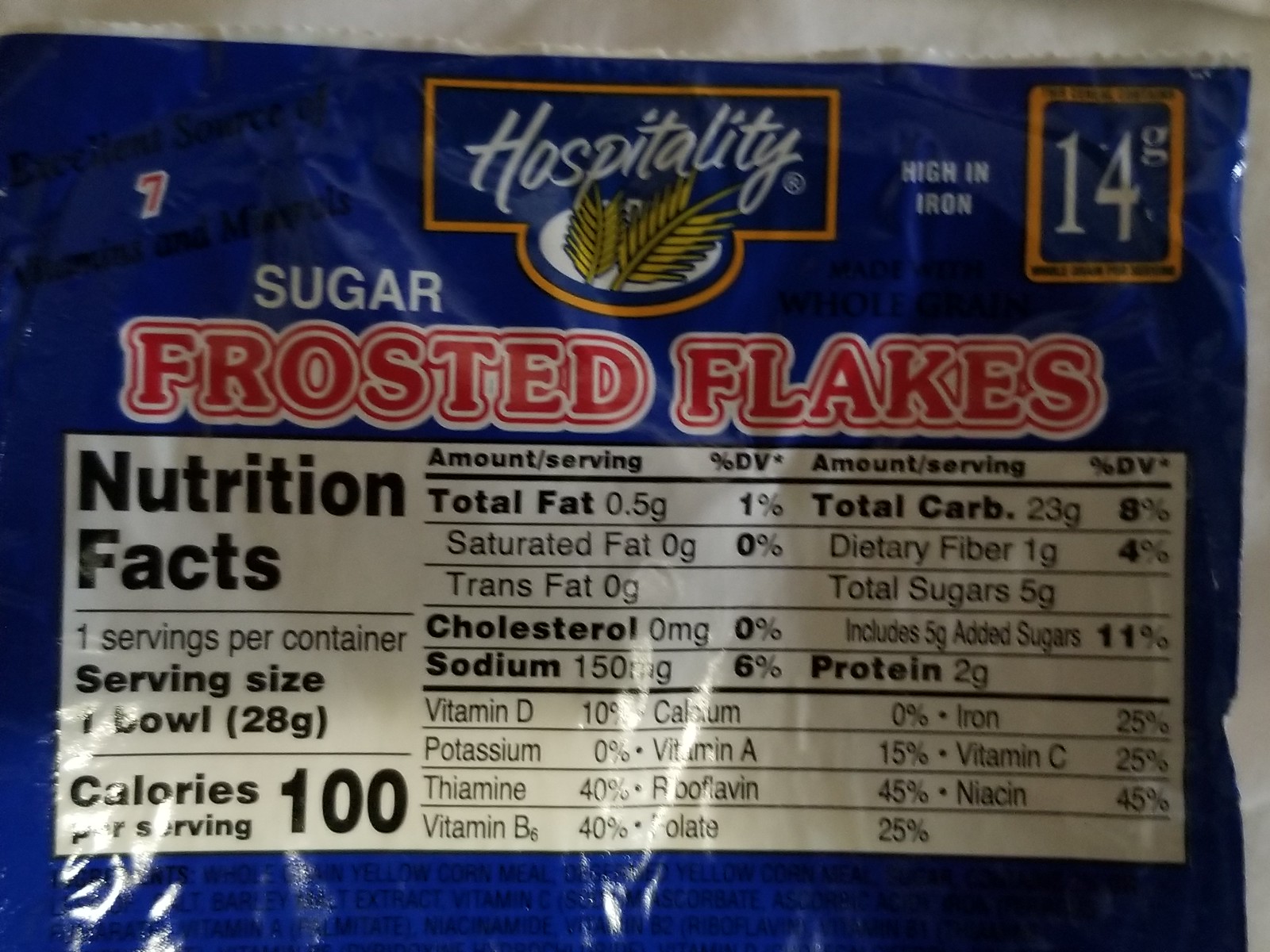The image depicts the food label of a product from the Hospitality brand. The label features the brand name "Hospitality" prominently inscribed in a cursive white font, accented by two yellow wheat shafts on either side of the logo. The logo is set against a rich blue background that is bordered with a gold trim, giving it an elegant and classic appearance.

This particular label is for Hospitality's "Sugar Frosted Flakes." The product name "Sugar Frosted Flakes" is clearly displayed on the label, indicating the item inside the packaging. The label also includes a Nutrition Facts section, which is presented in a black and white rectangular box. Outside of this Nutrition Facts box, additional notations emphasize the nutritional benefits of the product, highlighting statements such as "High in Iron" and "Excellent Source of Vitamins and Minerals," which are designed to attract health-conscious consumers.

The overall design and colors used on the label create a visually appealing and informative presentation, aligning with the brand's quality and reliability.